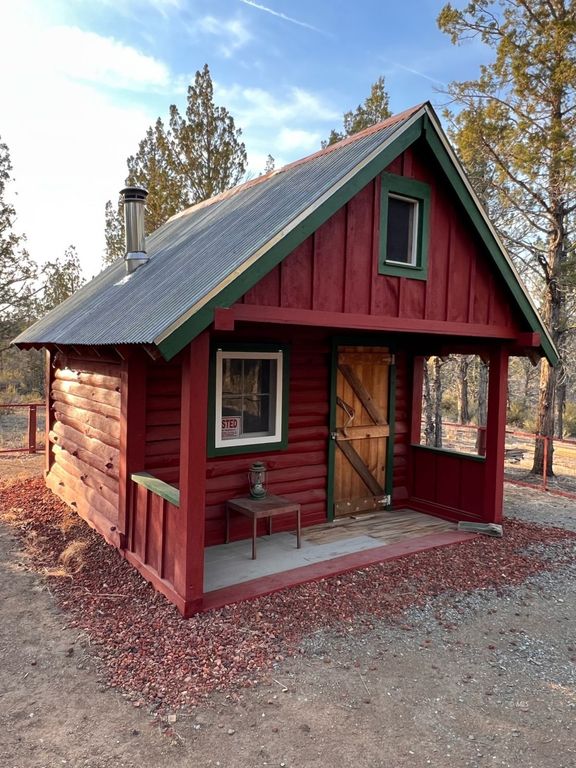This daytime photograph features a charming red wooden cabin, tucked away in a forested area. The cabin, resembling a small log shed, is adorned with a green triangular roof and matching green trim around its window and door. At the front, it boasts a quaint, shaded porch area where a small table holds a classic Coleman camping lantern. Above the lantern, a window displays a sign that appears to read "POSTED" in red and white letters. The door to the right of the window is made of unpainted brown wood, reminiscent of barn doors. A silver chimney stack emerges from the left side of the roof, hinting at a cozy interior. Encircling the cabin are tall trees, contributing to the serene forest setting, and a red fence can be seen extending around the back and sides of the cabin. The ground is covered in dirt and reddish mulch, with fallen leaves scattered near the edges of the structure. Above, the sky is a vivid blue, punctuated by fluffy white clouds, adding to the idyllic rural scene.